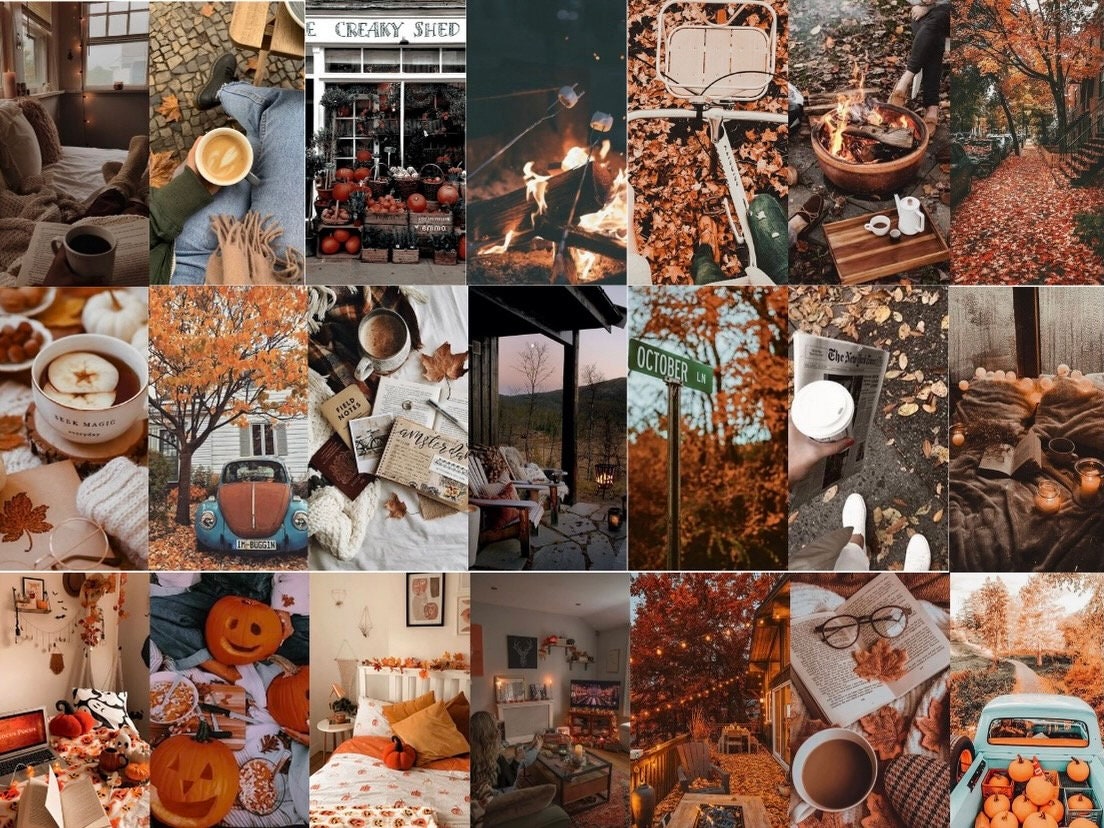A vibrant collage of fall-themed images captures the essence of autumn in vivid detail. The top row features a cozy scene with a steaming latte beside a person wrapped in a brown scarf, sitting near a bench. Adjacent to this, a charming 'Creaky Shed' fronts a display of pumpkins. Marshmallows roast over a fire in one image, while another shows a pile of wood burning brightly. The final image in this row showcases a sidewalk blanketed in orange, red, and yellow leaves, epitomizing the season's beauty.

The middle row continues the fall theme with a street sign reading 'October Lane,' set against a backdrop of brilliantly colored fall foliage. 

The bottom row includes a series of carved jack-o'-lanterns and a cozy bedroom adorned with autumnal decorations like leaf garlands on the headboard, orange pillows, and a pumpkin-shaped cushion. Nearby, string lights dangle from a porch overlooking trees bursting with fall colors, the porch itself blanketed in orange leaves. In the final image, a blue truck brimming with bold orange pumpkins drives down an autumn road, encapsulating the season's rustic charm.